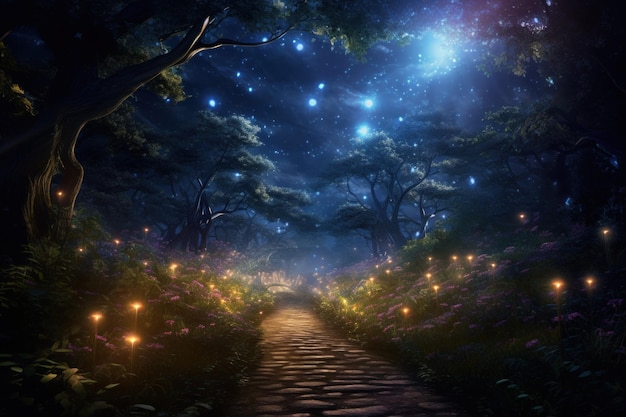In this photo taken at night, the scene exudes a mystical, almost fantastical ambiance. The night sky is abundant with stars of varying sizes, alongside a brilliant display of the Milky Way. The moon, partially veiled by the shadows of numerous trees, casts a reflective glow across the scene, illuminating a stone pathway that winds through the landscape. This pathway is flanked by small, enchanting lights and bordered by lush vegetation, including purple and white flowers interspersed with green leaves. Twinkle lights are artfully integrated throughout the garden, adding to the otherworldly atmosphere. The image’s rich, colorful palette of greens and blues contributes to its surreal quality, making it resemble a beautifully crafted piece from a video game or a fantasy movie. The presence of numerous tiny lights, which appear to be fireflies or candles, further enhances the enchanting feel of the scene, as they glow softly amidst the grass and undergrowth.